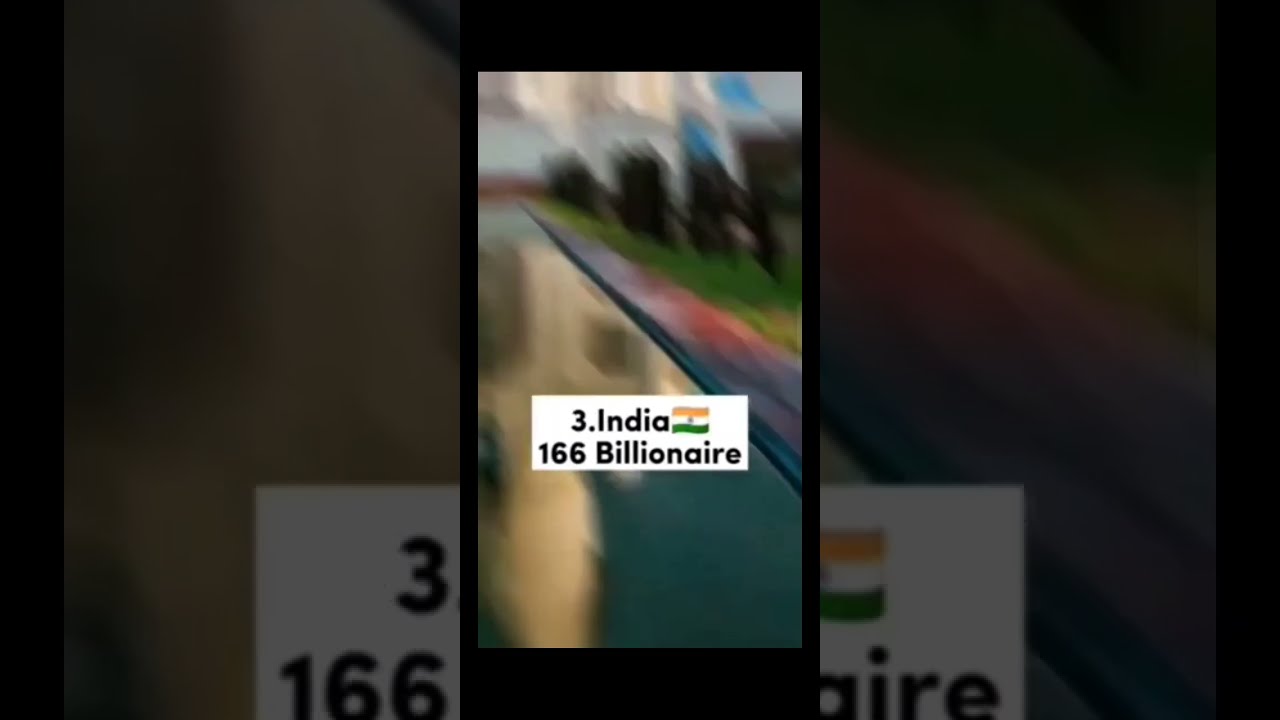This horizontal, rectangular image prominently features a vertical, rectangular cell phone screen at its center. Displayed on the cell phone screen is a white rectangle containing text in black lettering. The text reads "No. 3, India," followed by an Indian flag icon, and "166 Billionaire," with both "Billionaire" and "India" capitalized appropriately. The background of the image is a dynamic, blurry landscape with indistinct features suggesting green grass, tree shapes, and what might be a curb. Some parts of the background hint at a white structure with a pointy roof, possibly reflecting on a water surface, lending to the impression of a pool or body of water in the scene. The overall effect of the image is somewhat chaotic due to the extreme blur, making the detailed text box on the cell phone screen the focal point.